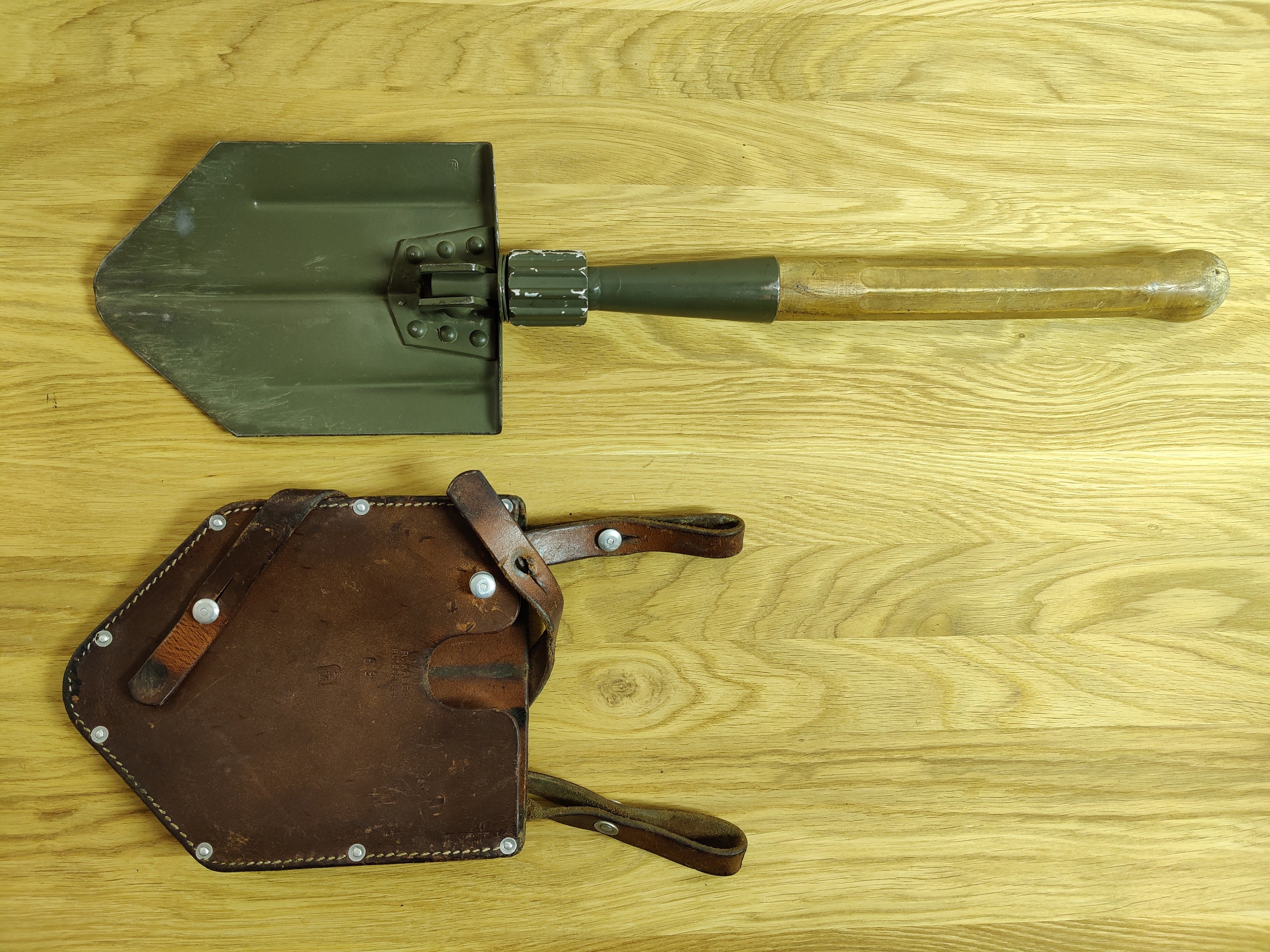The photograph showcases a classic military entrenching tool, commonly known as a shovel, laid out on a flat wooden surface. The wood, a light brown hue with distinct dark streaks of grain, serves as the backdrop for the well-worn tools. At the bottom of the image lies a leather sheath, pentagon-shaped with multiple buckles, clasps, and white stitching along its edges. The shovel itself, positioned above the sheath, features a metal head that can be adjusted or folded, exhibiting several scratches and dents indicative of extensive use. The metal spade, shaped like a pentagon and colored in a weathered green, attaches to a wooden handle about a foot and a half in length. A tightening knob beneath the spade adjusts its angle, allowing the shovel to be compacted for ease of transport. The leather sheath is designed to encase the spade, securing it for storage and protection.